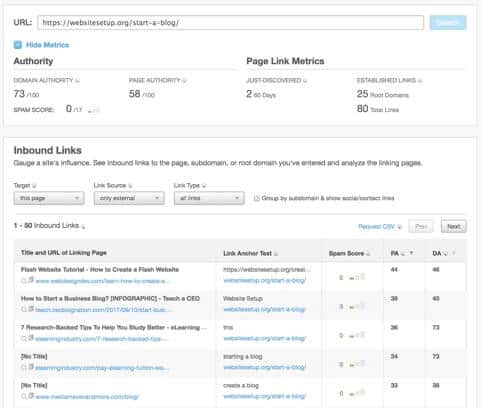This image captures a screenshot of a computer browser window, displaying the URL "website-setup.org/start-a-blog" prominently at the top. The screen features various metrics and statistics for a web page. Highlighted in blue at the top is the option labeled "Hide Metrics." Below, the screen is divided into sections with detailed information on page authority and links.

The "Authority" section indicates a score of 73 out of 100. Additional metrics include numbers 58, 2, 25, and 80, though their specific context is not immediately clear. Below this, there is a section for "Inbound Links," which is broken down further into "Target" specifying "This Page" and "Link Source" defined as "Any External." The "Link Type" section features the acronym "AT IBS."

The display continues with detailed breakdowns, enumerating "1 to 50 Inbound Links," presented in alternating rectangles of black and blue. Each blue section contains clickable link text. The pattern of black and blue rectangles extends down the page, with the sidebar also featuring similar link information. Each step of the webpage is meticulously color-coded and organized to convey detailed link metrics and authority ratings.